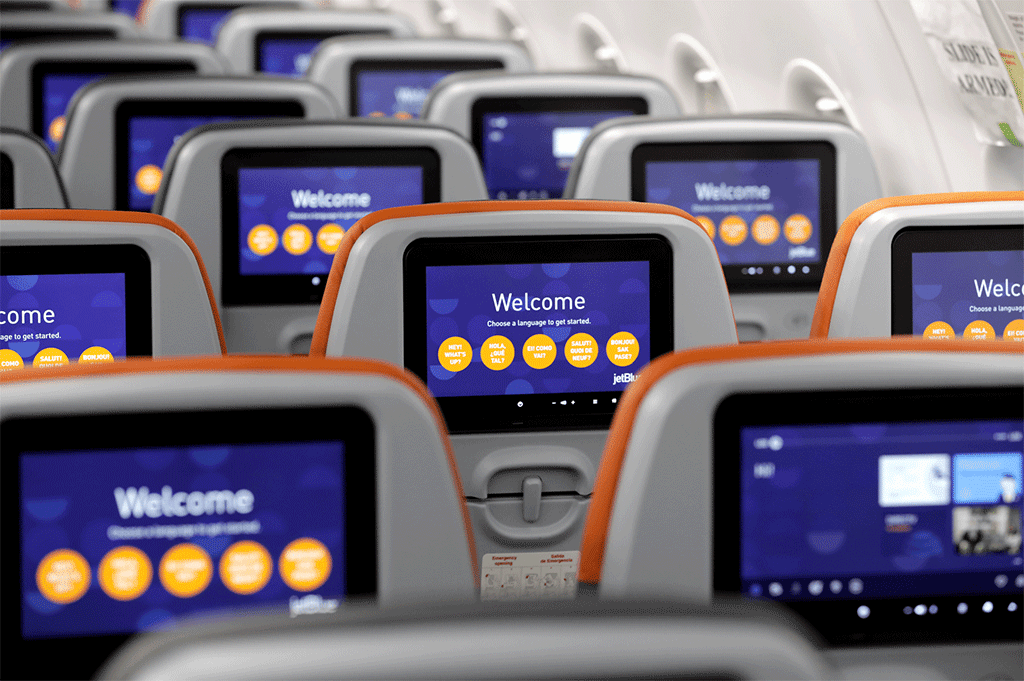This photograph captures the interior of a JetBlue airplane, focusing on several rows of passenger seats. Each seat is gray with orange trim and features a plastic frame. Prominently displayed on the back of every seat is a screen framed in black. The screens greet passengers with a "Welcome" message and prompt them to choose a language to proceed. Additionally, the screens, set against a blue background adorned with lighter circles and half-circles, feature five yellow interactive circles likely containing further information or options. The bottom right corner of each screen carries the JetBlue logo. Visible through the row of windows on the right side of the plane, an emergency instruction sticker is affixed to one of the seats, and a sign on the right wall reads "Slide is armed!" in bold black letters on white paper.